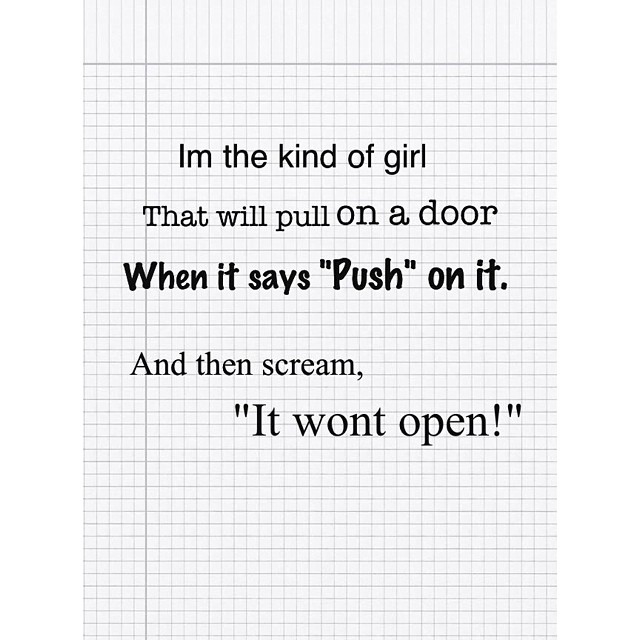The image features a white piece of graph paper with a light gray grid pattern, resembling lined graph paper but with a cartoonish, possibly illustrated or clip art appearance. The grid consists of many small squares, while the top eighth of the page displays only vertical lines, omitting horizontal ones. Superimposed on this backdrop is a lengthy, whimsically formatted text in varying shades of black and different fonts, ranging from thick to thin, Arial to Comic Sans. The text humorously declares, "I'm the kind of girl that will pull on a door when it says 'push' on it and then scream 'it won't open'!" with "push" and "it won't open!" emphasized in quotes. The word "won't" lacks an apostrophe, and the exclamation mark adds to the comedic tone. This playful font variation and the text's layout contribute to the quirky humor of the overall composition.